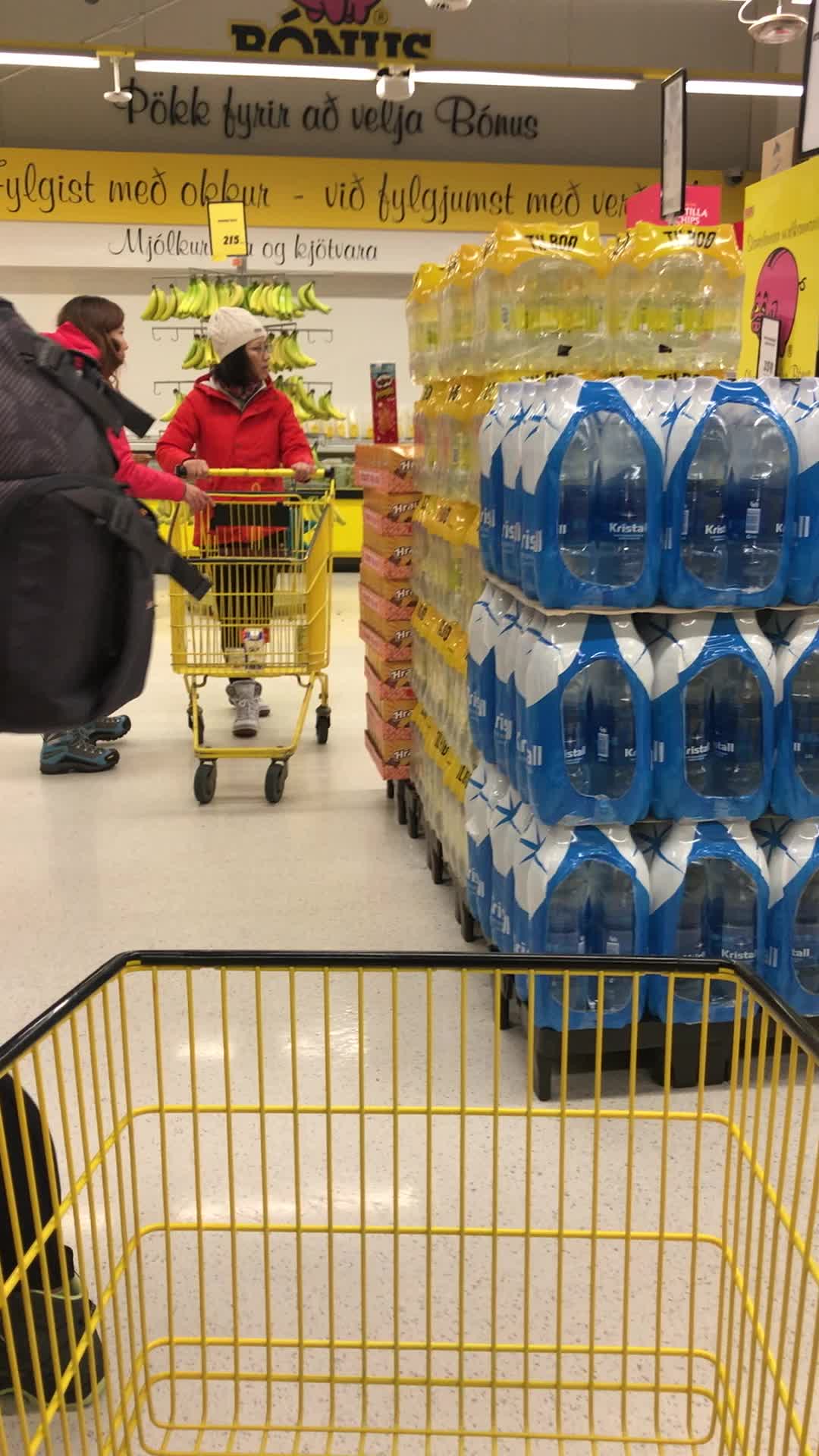The photo captures the interior of what appears to be a foreign supermarket, likely Vietnamese, as indicated by the non-English signage. In the foreground, prominently displayed is a yellow shopping cart with black trim around the top, seemingly being pushed by the person taking the photo. Straight ahead, there's another yellow cart being pushed by a woman in a red jacket, white winter hat, and gray shoes, with perhaps some small items at the bottom of her cart. To her left is another woman also in a red jacket, blue and black hiking boots, and medium-length brown hair. This second woman is looking off to the right of the image, while a black backpack partially obscures her body. 

Behind these women is a display of bananas, with a sign above it, various letters visible but ultimately unreadable due to the foreign script. In front of the banana display, there are stacks of bottled water, some in blue and white packaging, others in yellow, with the taller stack being yellow. A Pringles can rests on one of the stacks, which are displayed on plastic pallets. The scene is set against a floor of white-beige tiles. In the background, additional generic grocery store elements like shelves and fluorescent light fixtures blend into the ambiance of a typical supermarket.